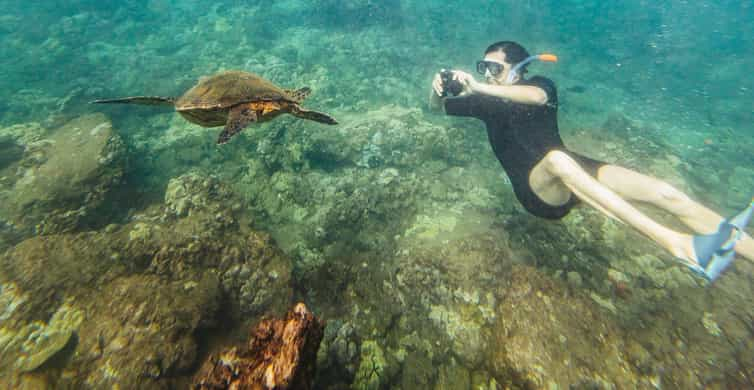In this vibrant underwater scene, a person wearing a short-sleeved black swimsuit and light blue flippers is captured mid-snorkel on the right. With black hair neatly secured under their goggles and an orange-tipped snorkel, they hold an underwater camera, aiming to photograph a striking green sea turtle swimming on their left. The sea turtle, seen from behind, exhibits a brownish-green hue as it gracefully glides amidst a diverse ocean floor. The seabed below is layered with various types of coral and rocks, showcasing a palette of earthy browns, mossy greens, and lighter shades of white and green, accentuated by the play of light through the blue-green water. An additional splash of orange coral adds a burst of color to this serene underwater tableau.